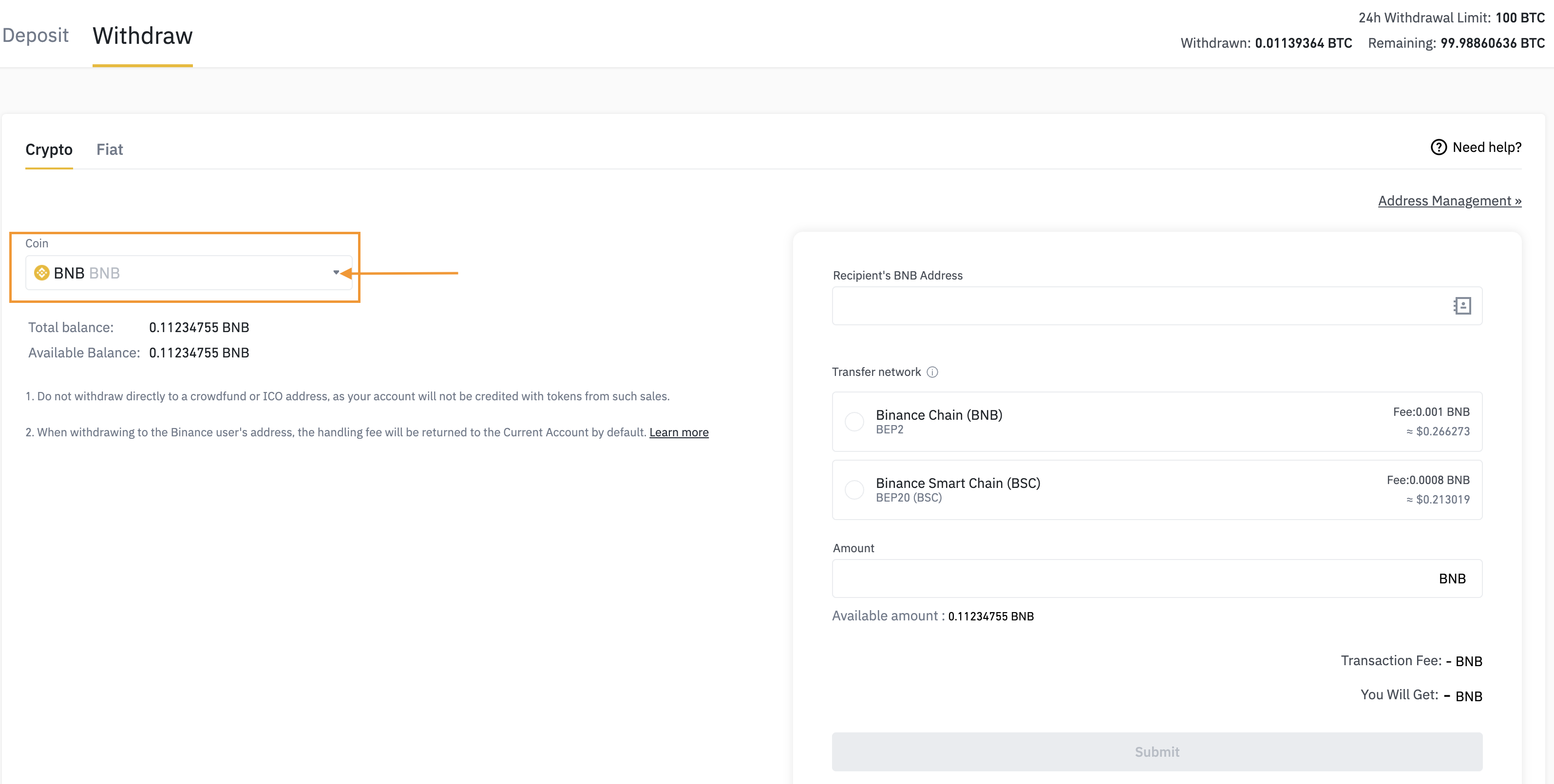Screenshot of BNB Bank's Website Interface:

The image captured showcases the interface of the BNB Bank's website, distinctly divided into two sections. On the left side, the primary focus is on the deposit and withdrawal functionalities. The 'Withdrawal' option is particularly emphasized, displayed in black font and highlighted with either a gray or gold bar beneath it. Directly below, there's a section dedicated to cryptocurrency activities, where specifics about a current crypto withdrawal attempt are visible. Here, users can observe their total balance, available balance, and helpful instruction notes for navigating the process effectively.

Contrastingly, the right side of the screen seems to be oriented towards transferring cryptocurrency to other users. This part includes detailed information about a recent transaction, albeit in very small and almost illegible font due to its size. The overall layout of the page is notably minimalistic, devoid of any distracting advertisements or banners. The design is sparse and functional, focusing solely on the essential details required for managing and transferring cryptocurrency between banks.